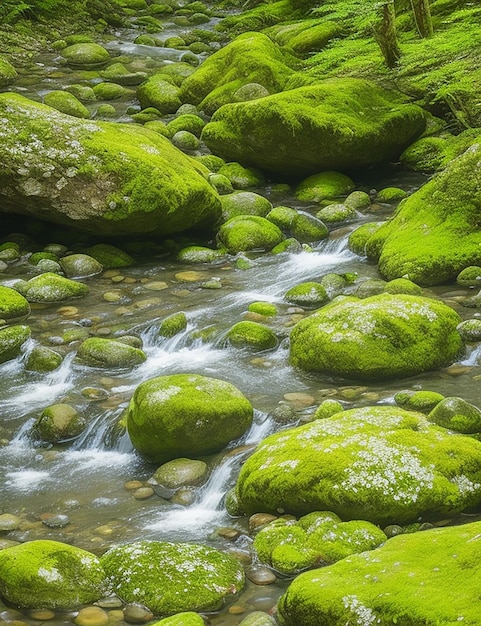A highly detailed and photo-realistic illustration captures a serene hillside stream meandering through a lush landscape of moss-covered rocks and boulders. Starting from the upper left quadrant of the image, the bubbling stream takes a zigzag path toward the right before veering back to the left. The majority of the stones and boulders are enveloped in vibrant green moss, contributing to the earthy palette of greens and browns that dominate the scene. Interspersed among the mossy rocks are delicate clusters of white to whitish-blue flowers, adding splashes of color to the verdant background. The flowing water, shallow yet dynamic, is aerated and frothy in sections, creating white caps that sparkle in the sunlight, suggesting a bright, sunny day. Subtle details like tree stems in the background hint at the proximity to a wooded area, enhancing the natural ambiance of this peaceful riverside scene.